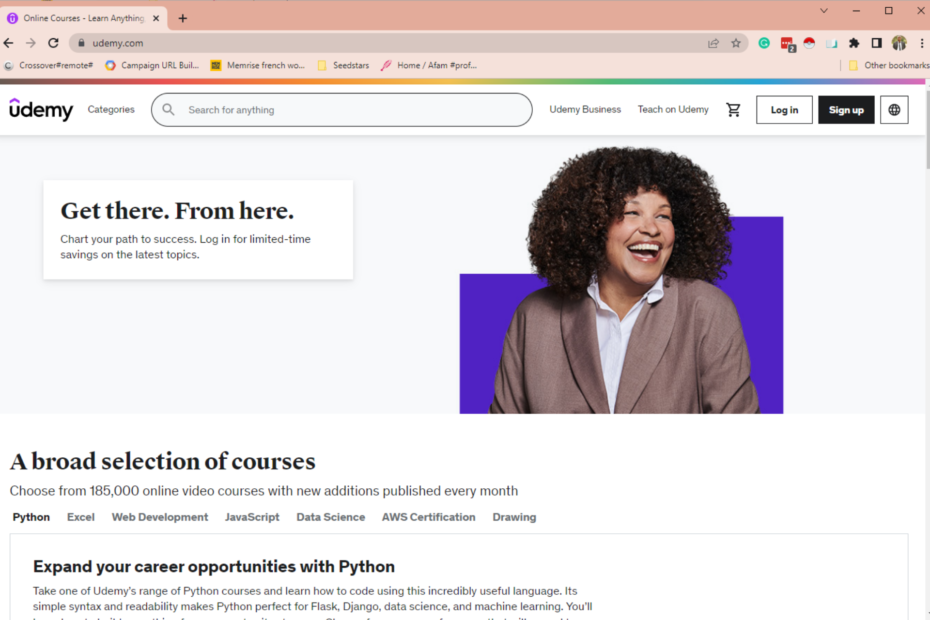This image is a detailed screenshot of a web browser displaying the Udemy website. 

At the very top, the application bar is visible, featuring the window buttons in the right-hand corner: minimize, maximize, and close. Beside these buttons is a downward-pointing arrow. On the left-hand side, there is an open tab showing the tab icon— a purple circle with a "U" underlined by a small hat-like figure— labeled "Online Courses - Learn Anything." To the right of this tab is a small "x" to close the tab and a plus symbol to open a new one.

Below the tabs, there is the navigation toolbar. It includes the back and forward buttons, a refresh button, and an address bar currently displaying "udemy.com." To the right of the address bar are several icons.

Beneath the address bar is a bookmarks bar containing a few bookmarked links: "Cross Over a More Remote Campaign," "Memorize French Words," "Seed Stars," and "Home/AFAM."

The main content of the webpage shows the Udemy site. The top left-hand corner features the Udemy logo, followed by a category label "Categories" and a search bar with the placeholder text "Search for anything." Adjacent to the search bar are links for "Udemy Business" and "Teach on Udemy," followed by icons for the shopping cart, login, sign up, and a globe indicating language selection.

Centered prominently on the page is an image of a woman looking to the side and laughing, accompanied by the text: "Get there from here. Chart your path to success. Log in for limited-time savings on the latest topics." Below this, there is a section titled "A broad selection of courses," stating, "Choose from 185,000 online video courses with new editions published every month."